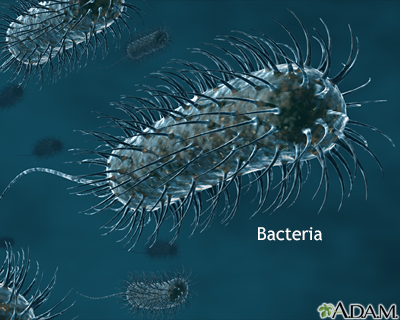The image depicts an intricate, close-up illustration of various bacteria against a dark, navy-blue background with a hint of teal. Centrally featured is a large, cylindrical bacterium, diagonally oriented, with a detailed, furry surface resembling thorns or spikes. This bacterium has a brownish-white body with blue tinges, much like a pill shape, and it possesses a long, flowing tail. Surrounding this central figure are smaller, similarly structured bacteria floating about, contributing to the dynamic scene. On the bottom right of the image, the word "Bacteria" is prominently displayed in white letters, while in the absolute bottom right corner, the text "Adam" (stylized as A.D.A.M.) is written in black. Additionally, a green flower-like logo is positioned on the left side of the image. The overall composition captures the minute and complex world of these microcellular organisms.